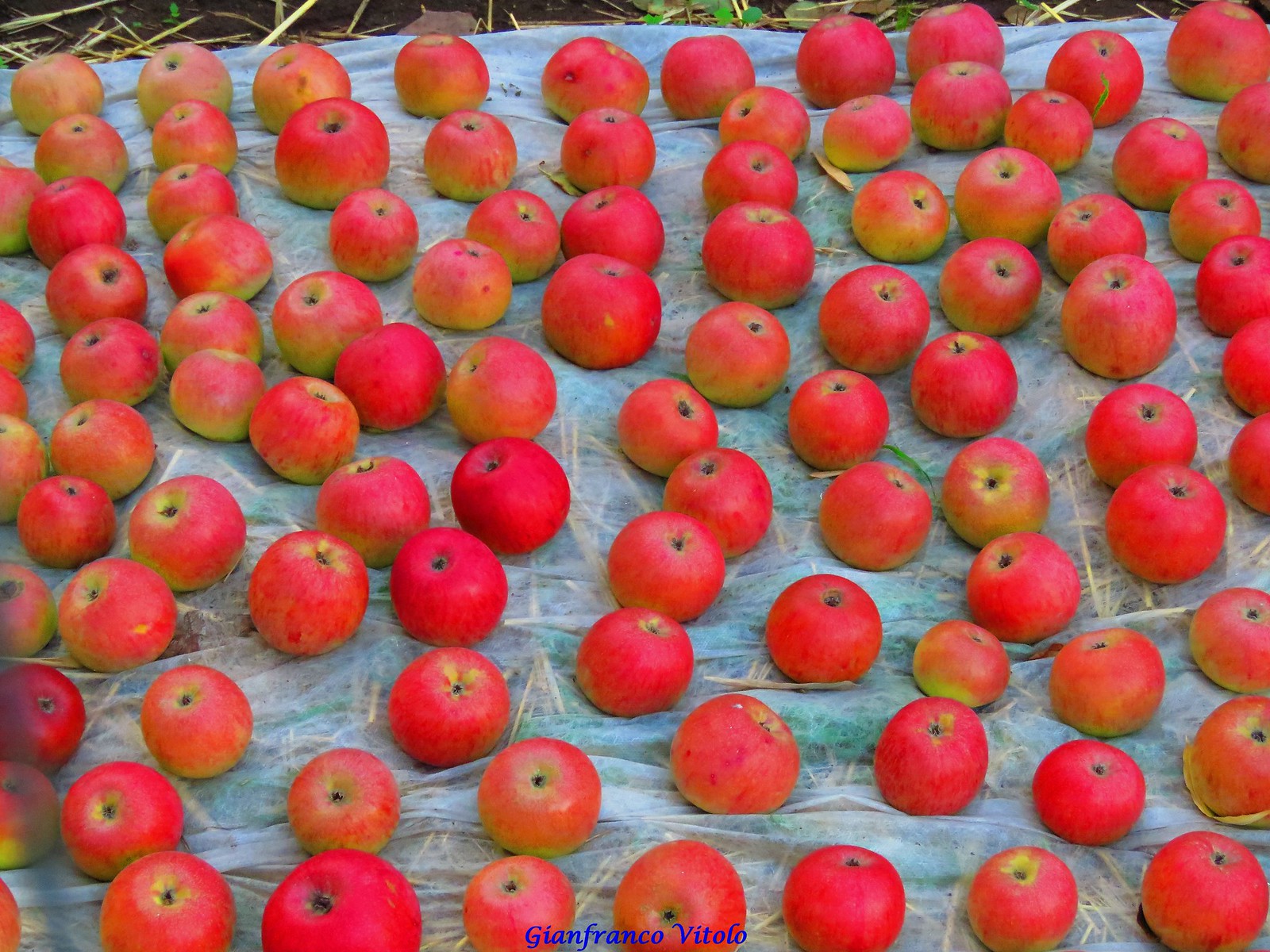The image is a vibrant color photograph showcasing an abundant spread of red apples that completely covers the frame. The apples are predominantly red with hints of green and some yellow patches around the stalks, which are mostly oriented upwards. They lie on a slightly curved, translucent blue hessian material that could be used for bundling the apples, possibly for sale at a farmer's market. Through this fabric, patches of brown grass or hay are faintly visible, suggesting an outdoor setting, potentially an apple orchard. Towards the back of the image, green leaves and shoots peek through, indicating the earthy surroundings. At the bottom center of the photograph, there's text in dark navy blue, capitalized as "GIANFRANCO VITOLO."